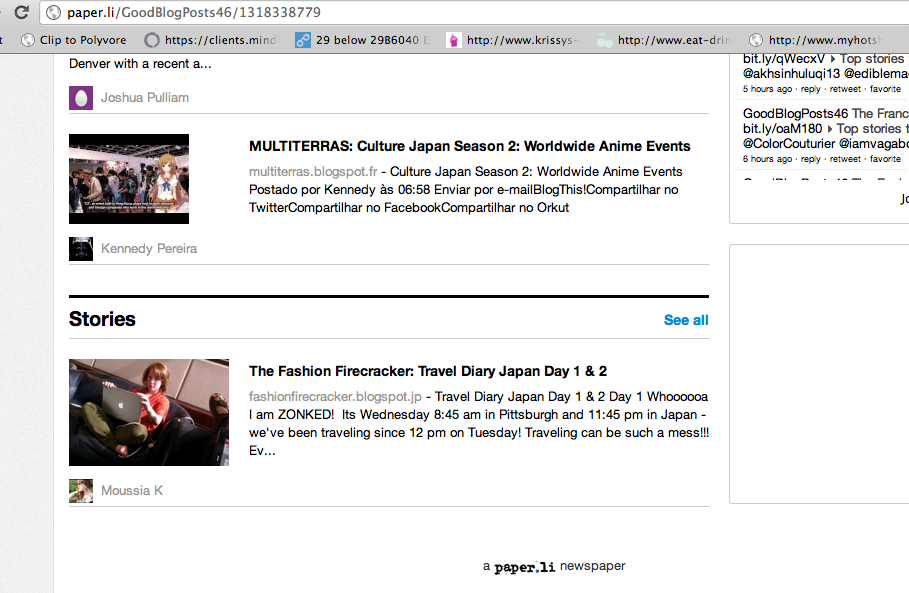The screenshot displays several blog posts featured on the website paper.li. The URL visible is paper.li/goodblogpost46/1318338779. The top navigation bar includes bookmarked items such as "clip to Polyvore," "clients.mind 29," and truncated titles like "Chrissy something" and "eat-drink." 

The forefront includes a partially obscured blog post from Denver that's been scrolled up, making it unreadable. Below this is a post by Joshua Pulliam titled "Multi Terra's Culture: Japan Season 2 Worldwide Anime Events," accompanied by an image of a crowd at a gallery or party with an anime character superimposed over it. 

Another post by Kennedy Pereira is visible, showing the title "Travel Diary: Japan Day One and Two" along with a black bar and call-to-action "story." An accompanying image depicts a woman, identified as "The Fashion Firecracker," sitting cross-legged in a round chair with a red Apple MacBook Pro. She has red hair and the context of the travel diary highlights the exhaustion from traveling. It mentions timestamps reflecting different time zones: 4:45 AM in Pittsburgh and 11:45 AM in Japan.

The top portion includes blurred or cut-off texts tagged as top stories with elongated URLs and perhaps social media elements, though their exact nature remains unclear. This screen capture is a representation of a paper.li newspaper, as noted at the bottom center. Overall, the screenshot appears visually cluttered and disorganized.